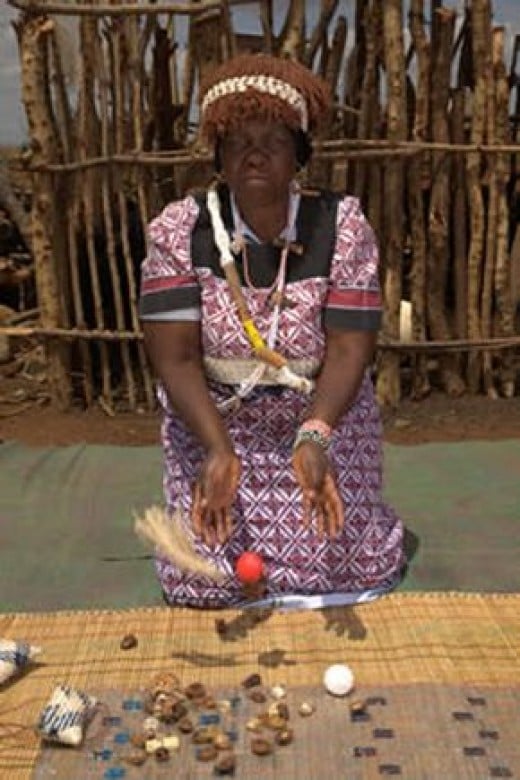In this image, we see an elderly African woman, possibly in her 60s or older, kneeling on the ground which is primarily dirt. The setting appears to be outdoors, possibly in a third-world country. The woman, centered in the photograph, has a rich brown complexion and is dressed in a beautifully patterned purple dress with geometric designs. On her head, she wears a woven hat with a white band, and she is adorned with necklaces made of woven materials.

She has an upset expression, her hands extended over her lap. Between her hands, in midair, is a small red ball, appearing as if she is tossing it. In front of her lies a woven mat dotted with small objects, including stones or beads, as well as a small white ball and the red ball she’s tossing.

Behind her stands a rustic fence, composed of tall branches standing vertically with additional sticks connected horizontally, creating a crude but functional barrier. The image includes a variety of colors, including brown, gray, white, pink, purple, yellow, orange, and dark blue, adding to the vividness and texture of the scene. The overall atmosphere suggests a quiet, solitary moment captured amidst simple yet intricate surroundings.